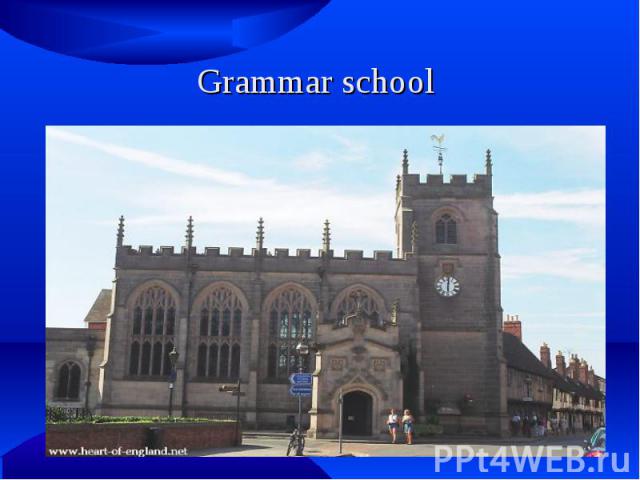The photograph titled "Grammar School" prominently displays the words "Grammar School" in white letters across the top within a blue border, which varies in thickness. Beneath the title is an image of a large, stone building resembling a cathedral or church, suggesting it may have served as a grammar school. The building features a tower with a clock and several tall, arched windows with vertical bars. A weather vane sits atop the tower. The structure is primarily grayish-brown stone with a dark brown door to the left of the tower, and two women are posing near the entrance. The scene is illuminated by sunlight under a blue sky with long, thin white clouds. In the lower left corner of the image, just above the border, the website "www.heartofengland.net" is visible, while the lower right corner features "ppt4web.ru," indicating some involvement with Russia. To the right of the church-like structure, a London street stretches out, hinting at its possible European location.